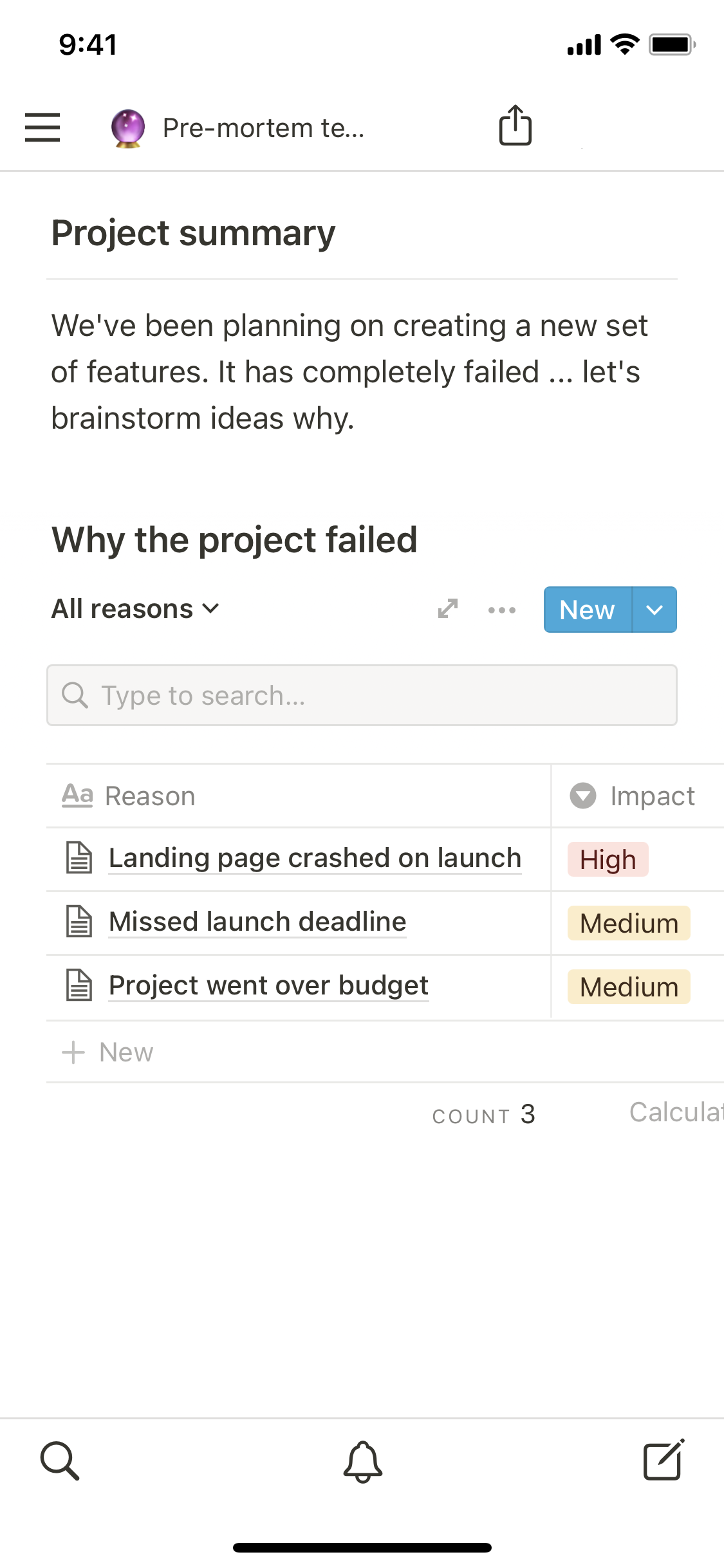A detailed caption for the image described could look like this:

---

The image is a screenshot taken from a smartphone, showcasing a white background. In the upper left-hand corner, the time is displayed as 9:41. Moving to the right, the top bar includes signal bars, a Wi-Fi connectivity icon, and a fully charged battery icon, depicted as a black-filled horizontal battery symbol. Below the top bar, there are three horizontal gray lines next to a purple crystal ball icon accompanied by the text "pre-mortem te..." and an adjacent upload button. Below this, a faint green horizontal line is visible, leading down to a "Project Summary" section. Beneath this, another even fainter green line stretches horizontally, and the text reads: "We've been planning on creating a new set of features. It has completely failed. Let's brainstorm ideas why." As the viewer scrolls down, they encounter a section titled "Why the project failed," with a search bar labeled "All reasons" for input. To the right, there is a blue "New" button. Listed reasons for the project's failure include: "Landing page crashed on launch" marked as high with red color, "Missed launch deadline" and "Project went over budget" both marked as medium with yellow color.

---